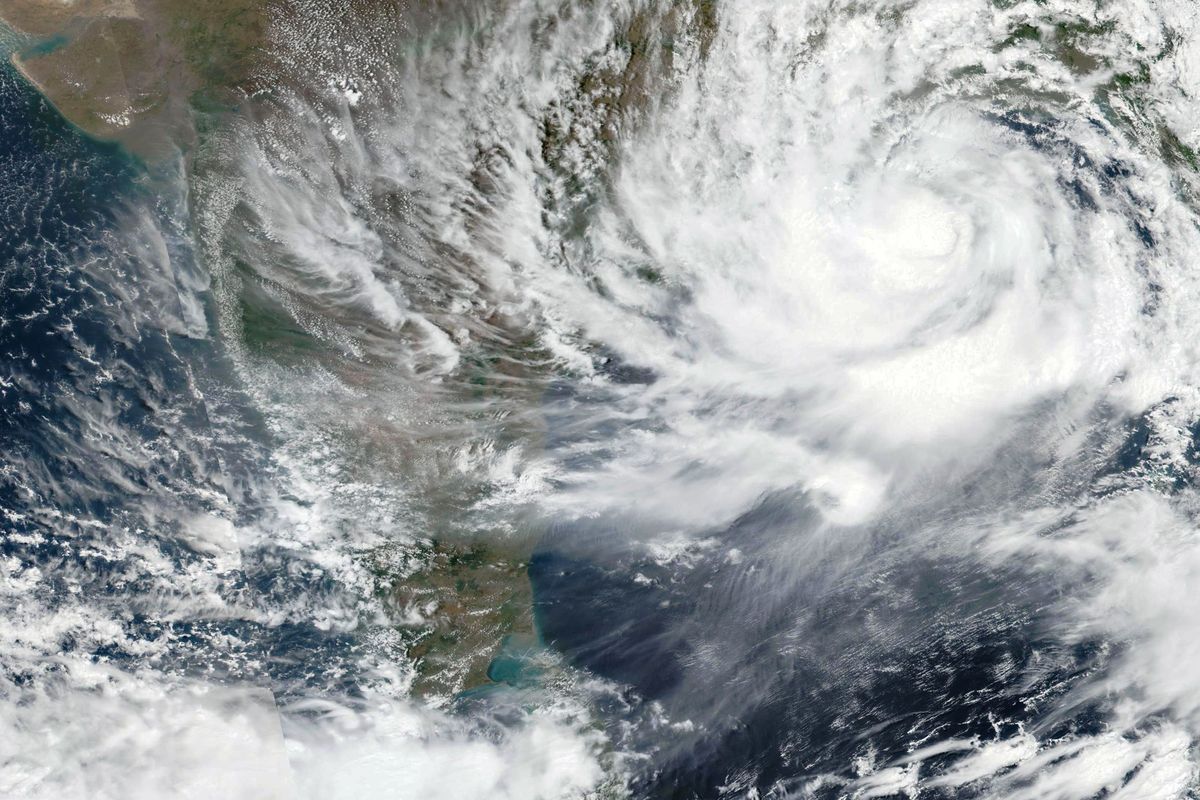This captivating satellite photograph, oriented horizontally, captures a dramatic aerial view of a massive hurricane swirling over the ocean. The eye of the hurricane, a calm and circular region, sits prominently in the upper right portion of the image, surrounded by dense, white, swirling clouds that form a striking vortex. This powerful weather system appears to be on the verge of making landfall, with an expansive and diverse landmass visible along the left side of the image. The land, characterized by brown and green hues, tapers towards the bottom, allowing the deep, dark blue of the ocean to reappear in the lower left corner. The tumultuous waves and white foam accentuate the dynamic interaction between the storm and the ocean, painting a vivid and somewhat ominous scene from a vantage point high above Earth.